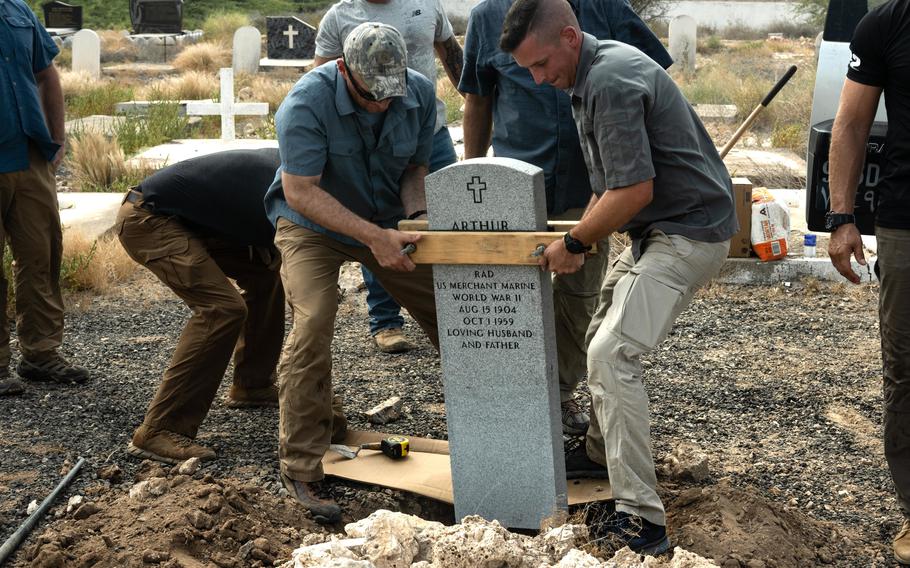In this highly detailed, color photograph set in a cemetery, two strong, military-type men are carefully positioning a tall, vertical gray tombstone with a slightly rounded top and a black outline of a cross at the peak. The name "Arthur" is prominently engraved on the tombstone, which commemorates a World War II veteran. The men are on either side of the tombstone, each holding a wooden plank to stabilize it as they place it into a freshly dug hole surrounded by white rocks.

On the left, a man wearing a blue short-sleeve button-down shirt and a camo hat grips the wooden board firmly. The man on the right, with a sharp military haircut, is dressed in a dark gray shirt and beige long cargo pants, mirroring the attire of his counterpart. Surrounding the scene are additional men, indistinct but similarly dressed in brown pants and blue shirts, engaged in various tasks related to the grave setting. Background details reveal multiple tombstones with crosses, reinforcing that the scene is taking place in a cemetery. This photograph captures the solemn and meticulous process of grave marking, embodying photographic representational realism.